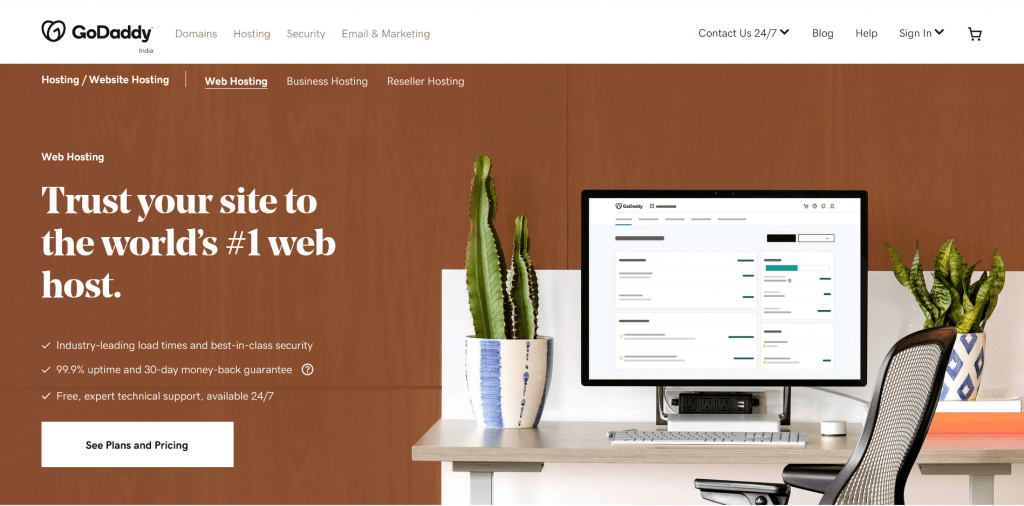The image is a screenshot of the GoDaddy India website. The GoDaddy logo, along with the word "GoDaddy" next to it, is prominently displayed in the upper left corner. Directly below the logo, in small grey letters, it reads "India," indicating this site is tailored for Indian users.

Across the top of the page, there is a navigation menu with the following categories in light grey text: "Domains," "Hosting," "Security," "Email," and "Marketing." Towards the right side of the menu, it includes options for "Contact Us 24x7" with a drop-down icon, followed by "Blog," "Help," "Sign In" (also with a drop-down icon), and a shopping cart symbol.

The background of the image shows a cozy office setting with brown walls or paneling. Central to this setting is a desk monitor, situated on a light brown-colored desktop which could either be made of wood or pressed wood. On either side of the monitor are two plants: the plant on the left is in a blue-and-white, vertically striped planter and resembles a tall cactus, while the plant on the right is in a blue-and-white planter decorated with small blue diamonds, hosting what appears to be a fern or leafy plant with semi-tall leaves.

On the left side of the page content, there are navigation links for different hosting services, including "Website Hosting," which is currently highlighted and underlined in white, "Business Hosting," and "Reseller Hosting." The main section reads "Web Hosting" in large white letters, with a compelling tagline underneath: "Trust your site to the world's number one web host."

Further details include smaller white text that highlights GoDaddy’s key features: "Industry-leading load times and best-in-class security," "99.9% uptime and 30-day money-back guarantee," and "Free expert technical support available 24-7," each marked with a white tick on the left. Beneath these features, a clickable white rectangle with black text says, "See plans for pricing."

Below the monitor, the desk also holds a keyboard directly in front and a white mouse to the right. The chair facing the desk is turned slightly to the left and sports armrests, made of black or dark gray material, with a mesh design for the backrest. There are no additional images or text, making it clear that this screenshot captures the essence of the GoDaddy India website’s web hosting page.